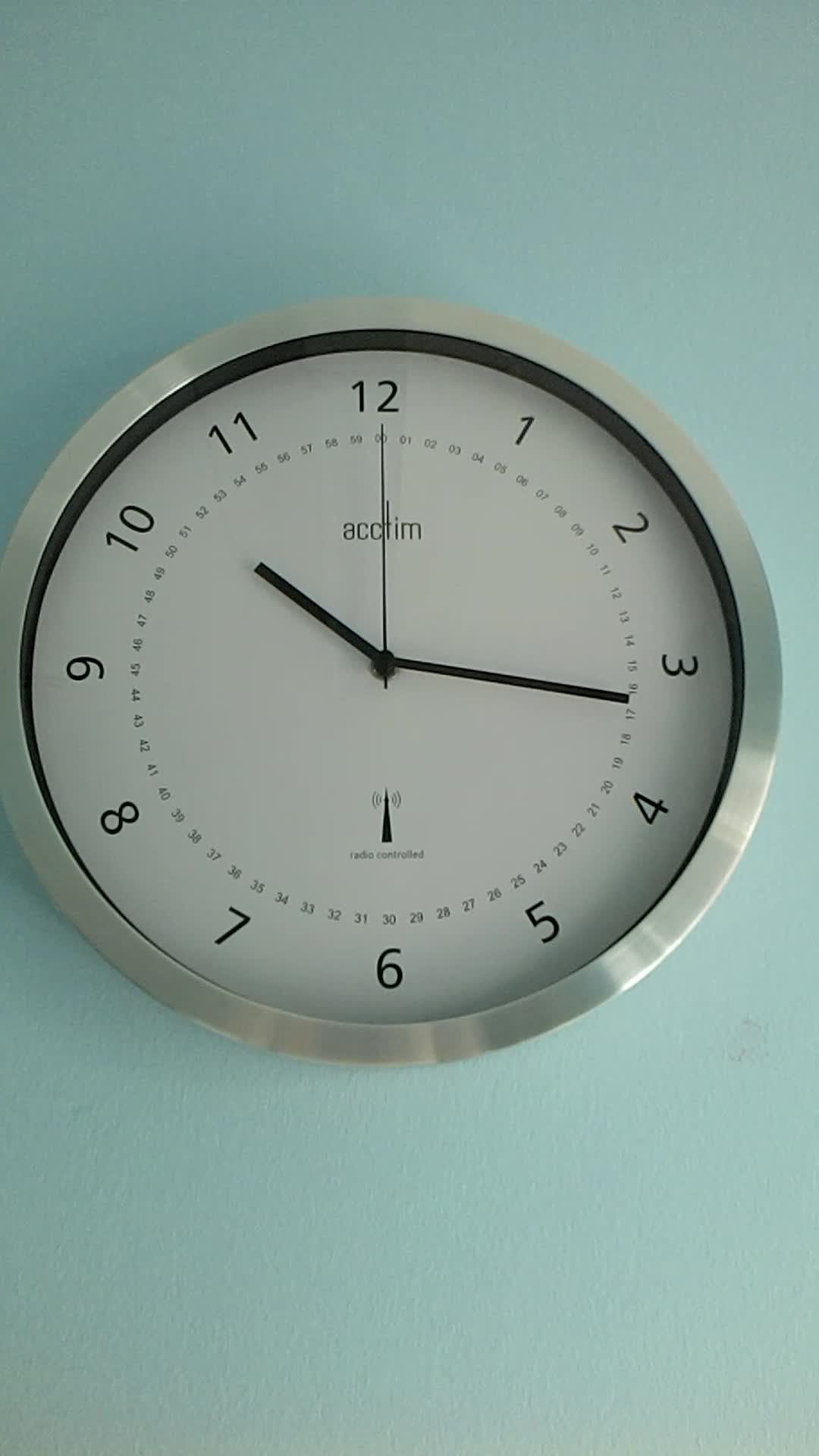The image is of a round wall clock positioned on a pale blue background. The clock has a silver metal trim that reflects light, adding depth to its appearance. The face of the clock is white with large, easy-to-read numbers from 1 to 12, marked for the hours. Additionally, there is a separate inner ring with smaller numbers indicating the minutes or possibly seconds. 

The time displayed is 16 minutes past 10, with the thin second hand pointing straight up at the 12. Just below the 12, the clock bears the brand name "Actim" and features a graphic resembling a triangle. Underneath this logo, in small text, it says "Radio Controlled". There is also a small black line and additional text that's too tiny to read.